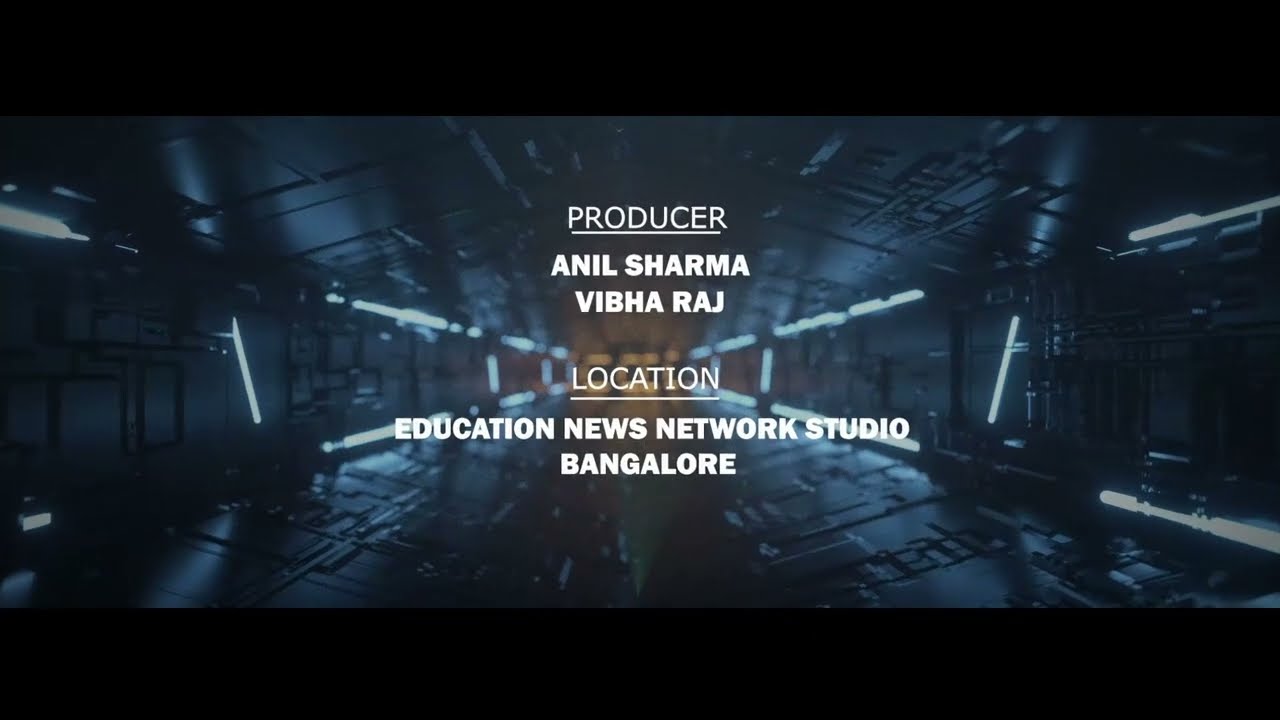The image is a letterboxed screenshot of what appears to be movie or television credits displayed on a dark, futuristic sci-fi corridor. The corridor resembles an interior of a spacecraft or perhaps a scene from a video game reminiscent of Star Wars, complete with high-tech metallic floors and ceilings accented by white neon lights lining the passageway. The focus of the image is a centered block of white text in six rows: the first row reads "PRODUCER" underlined, followed by the names "Anil Sharma" and "Vibha Raj." After a small space, the word "LOCATION" is underlined, followed by "Education News Network Studio" and "Bangalore."